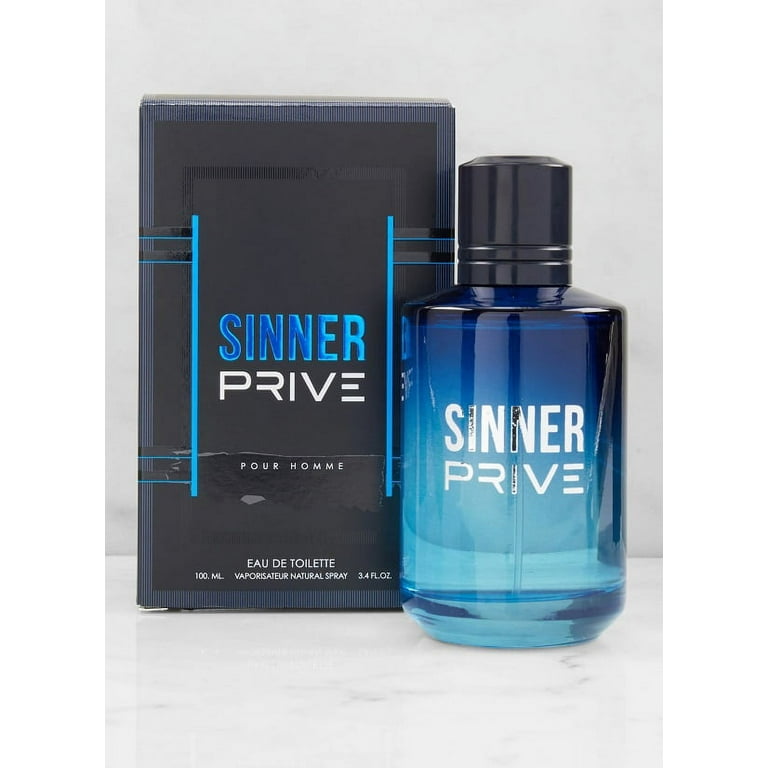The image features a men's cologne product presented on a grey backdrop, likely intended for a sales advertisement. On the left side is a sleek black rectangular box with glossy electric blue highlights. Centered on the box, "SINNER" is prominently displayed in vibrant blue letters, followed by "PRIVE" in a distinct white cybernetic font. Below this, in white text, the box reads "Pour Homme," and at the bottom, "Eau de Toilette," along with the details: "100 milliliters, 3.4 fluid ounces, vaporisateur natural spray."

Adjacent to the box, slightly in front, the cologne bottle itself shares the spotlight. The bottle has a striking blue gradient, transitioning from a dark blue at the top to a lighter blue at the bottom, giving it a teal appearance. The center of the bottle features the same "SINNER PRIVE" labeling in white text, and the bottle is capped with a black twist top. The liquid inside appears clear. Both items rest on a grey marble table, complementing the overall sophisticated presentation.